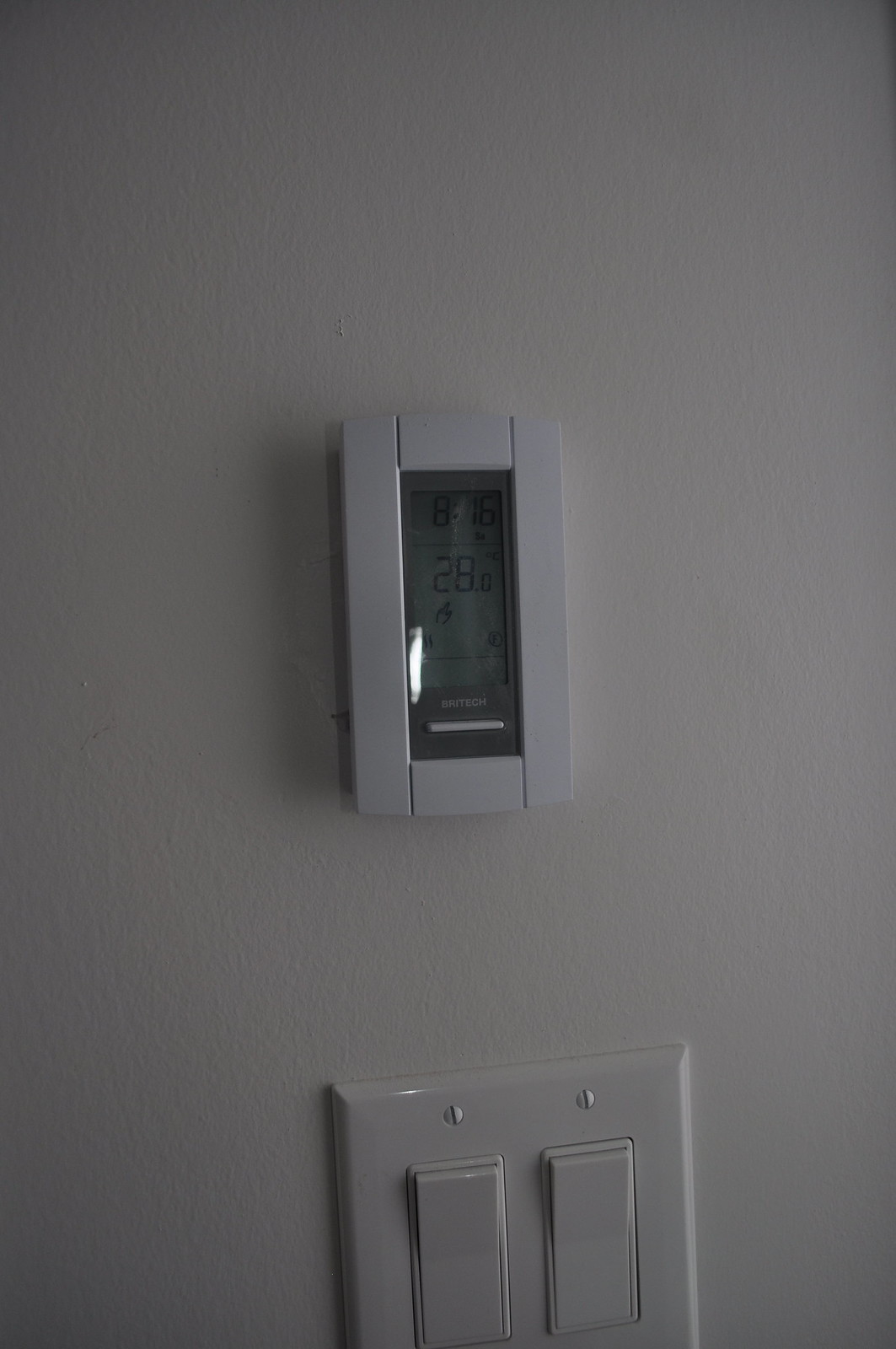In the center of the image, a digital thermostat is mounted on a wall, a bit distant and shrouded in dim lighting, making it somewhat difficult to read. The thermostat's digital display shows a temperature of 28.0 degrees, likely in Celsius. Above the display is a clock indicating the time as 8:16. There are several small, unclear marks below the display, which are too tiny to identify. The brand name appears below the digital display, but the text is not legible other than containing the word "tech." The thermostat has a gray background with white text and is bordered by a white frame. Below the thermostat, two flat, thick light switches are visible, designed to be pressed either on the top or bottom portion to operate.